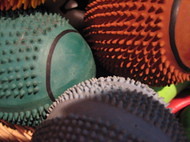The image is a close-up photograph of three spiky rubber dog balls, each a different color, and arranged together in a small rectangular frame. The ball in the foreground is purplish and partly shrouded in shadow, giving it light and dark purple hues. It features small, soft rubber nodules and a distinct black stripe around its center. To the left, there is a green ball that appears more of a teal or faded green shade. Like the other balls, it has spiky projections and a smooth central band marked by a black circular line. The ball on the right is an orangish-reddish or rust color, with the same spiky texture and black stripe. The lighting highlights the green and orange balls, whereas the purple ball remains partially shadowed. There are glimpses of other colorful objects, possibly other toys, in the background, adding bright hints of green, red, yellow, and blue.